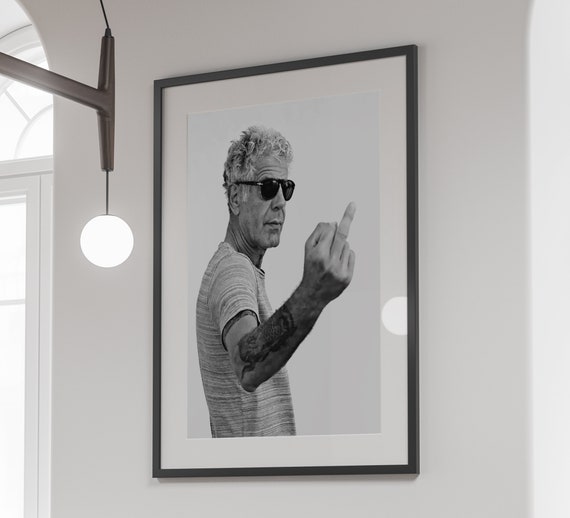This black and white photograph, measuring approximately four feet high by three and a half feet wide, is presented within a black frame with a white mat and hangs on a white wall. It depicts the renowned chef Anthony Bourdain, captured in profile with a serious expression, graying curly hair, and wearing dark aviator sunglasses. Bourdain, dressed in a light-colored T-shirt with fine horizontal stripes and a visible tattoo on his right forearm, is prominently shown giving the middle finger with his right hand. The monochromatic photo within the frame is set against a larger white piece of paper. To the left of the photo frame, a ceiling-mounted light hangs down from a steel beam by a pulley, casting a reflection on the right side of the frame. Adjacent to the picture is a white door with clear glass panels and a bent glass skylight, allowing natural light to spill into the space. The right edge of the setup includes a sliver of a doorway, adding depth to the scene.